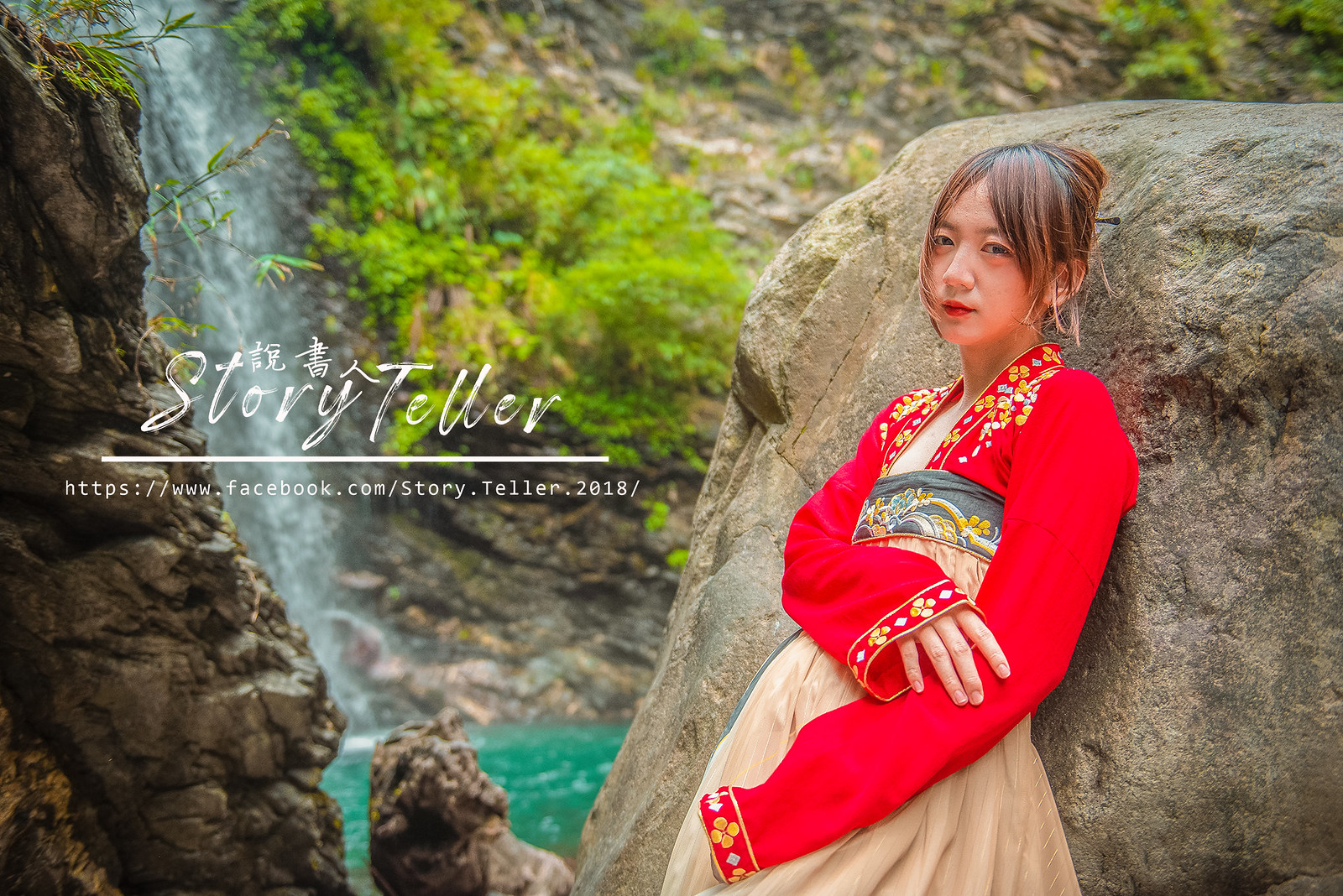The image features a woman leaning against a large rock with a scenic waterfall and rocks surrounded by green plants in the background. She is wearing an older-fashioned dress with very long red sleeves adorned with cuffs that have floral-like patterns in yellow, white, and gray, as well as white diamond shapes. The top part of her dress is red with a gray sash, and the bottom part is tan. Her hair is styled up, and her right hand rests on the inside of her left elbow. On the left side of the image, there is white text that says "Storyteller," followed by a line and a website URL, "https://www.facebook.com/story.teller.2018/," printed in smaller white letters below the line.